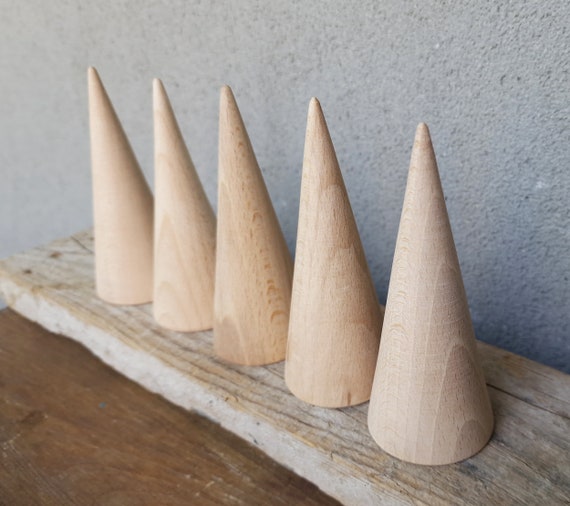The image depicts five pointy wooden cones meticulously arranged side by side on a weathered, light brown wooden board. The board itself rests atop a darker wooden support structure, creating a harmonious contrast between the varied shades of brown. Each cone is cylindrical at the base, tapering smoothly to a sharp point, and their surfaces reveal intricate circular patterns akin to growth rings, suggesting they were crafted on a lathe. Notably, the third cone from the left is distinguished by a dark, elongated circular occlusion near its base. The backdrop features a textured concrete wall, with a rough, "popcorn ceiling"-like finish that transitions from dark gray on the right to a lighter gray on the left. The careful alignment and uniform color of the cones, which resemble a pale sand hue, further underscore the craftsmanship and aesthetic appeal of the composition.